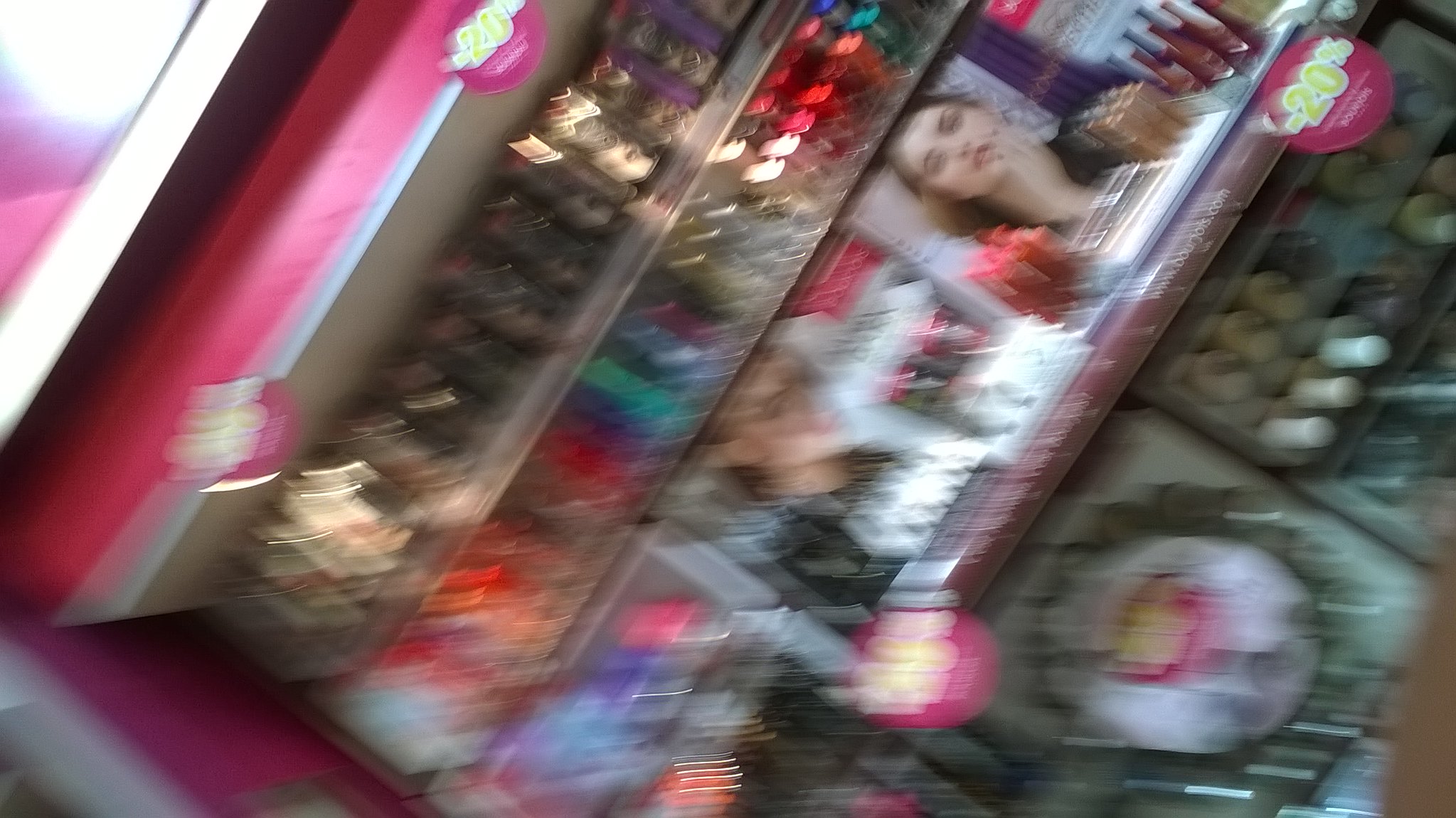The image is a very blurred photograph taken from a diagonal perspective, slanting up towards the right corner, capturing a bright and colorful cosmetics display in a store. The shelving framework, characterized by a bright pink color with silver accents, features four rows crowded with various vibrant products. The items on display include tubes, possibly containing personal care or cosmetic products like lipstick, lip gloss, nail polish, and eyeliners, arranged in color groupings of gold, brown, purple, pink, and white. The top left corner of the frame includes a white circular shape, while pink rectangles and silver lines are discernible below. The bottom row appears to contain larger items, and there are pink stickers with "20% off" written in yellow attached to the edges of the shelves. Additionally, the third row displays a blurred image of a woman, suggesting a model advertising the beauty products, with her makeup prominently featured. The composition is tilted to the right, creating an off-kilter view of the shelf against a predominantly pink and silver display background.